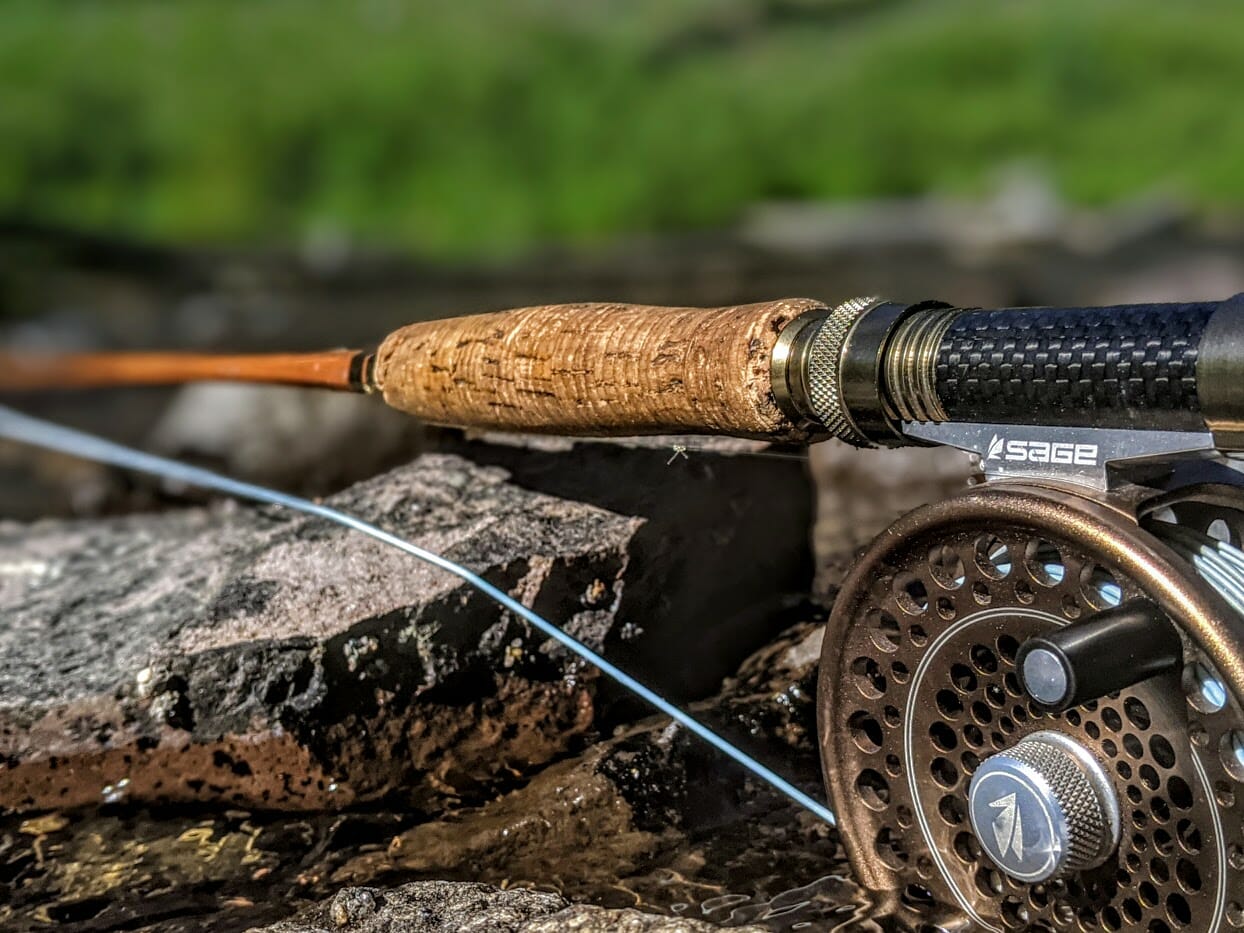The image showcases a close-up advertisement for a SAGE fishing rod. The rod is laid out on damp, grayish rocks with some greenery blurred in the background, suggesting an outdoor setting. Focused on the handle and reel, the SAGE trade name is prominently displayed. The handle sports a black textured grip with a leather-like inlay for comfort, transitioning to a brass or gold attachment. Moving forward, the handle is encased by a cork-like tan material, followed by the thin brown rod. Highlighted in the right corner is the bronze flywheel, adorned with the SAGE logo and a small black handle, with yellow and light blue fishing lines extending from the reel.